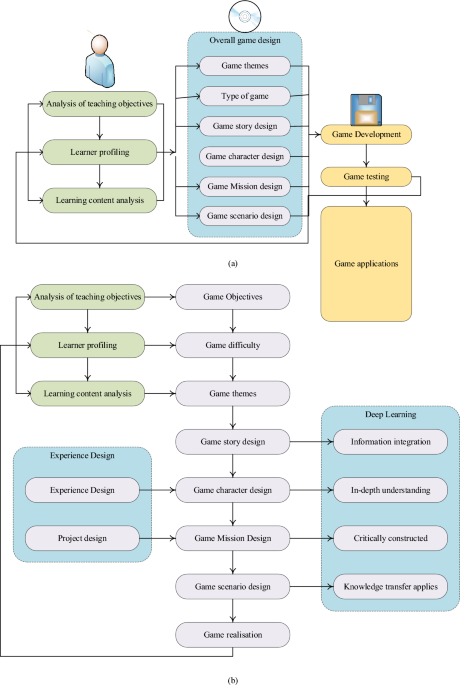The image is a vertically oriented diagram composed of two complex flowcharts related to game design and education. The upper flowchart focuses on overall game design and development, featuring three main columns interconnected by black lines and arrows. At the top center, boxes detail various aspects of game design such as Overall Game Design, Game Themes, Types of Game, Game Story Design, Game Characteristics, Game Mission, and Game Scenario. The left column highlights the Analysis of Teaching Objectives, Learner Problems, and Learning Constant Analysis, all feeding into the central column of game design aspects. To the right, the flowchart continues with Game Development, Game Testing, and Game Applications, leading to a small box symbolizing the final game.

Beneath this, the second flowchart delves into educational objectives and deep learning. The left column displays Analysis of Scaling Objectives, the center focuses on Game Objectives, and the right touches on Deep Learning. These components interconnect, suggesting an integrated system designed to create a learning experience through the game.

The diagram's dominant colors are white for the background, with elements in light blue, green, and light gray. Iconography includes a floppy disk and a 3D axonometric figure resembling a person, likely signifying the human element in game design and educational interaction. Overall, the image illustrates a multi-stage process aimed at developing an educational video game for students, emphasizing both game design and teaching objectives.